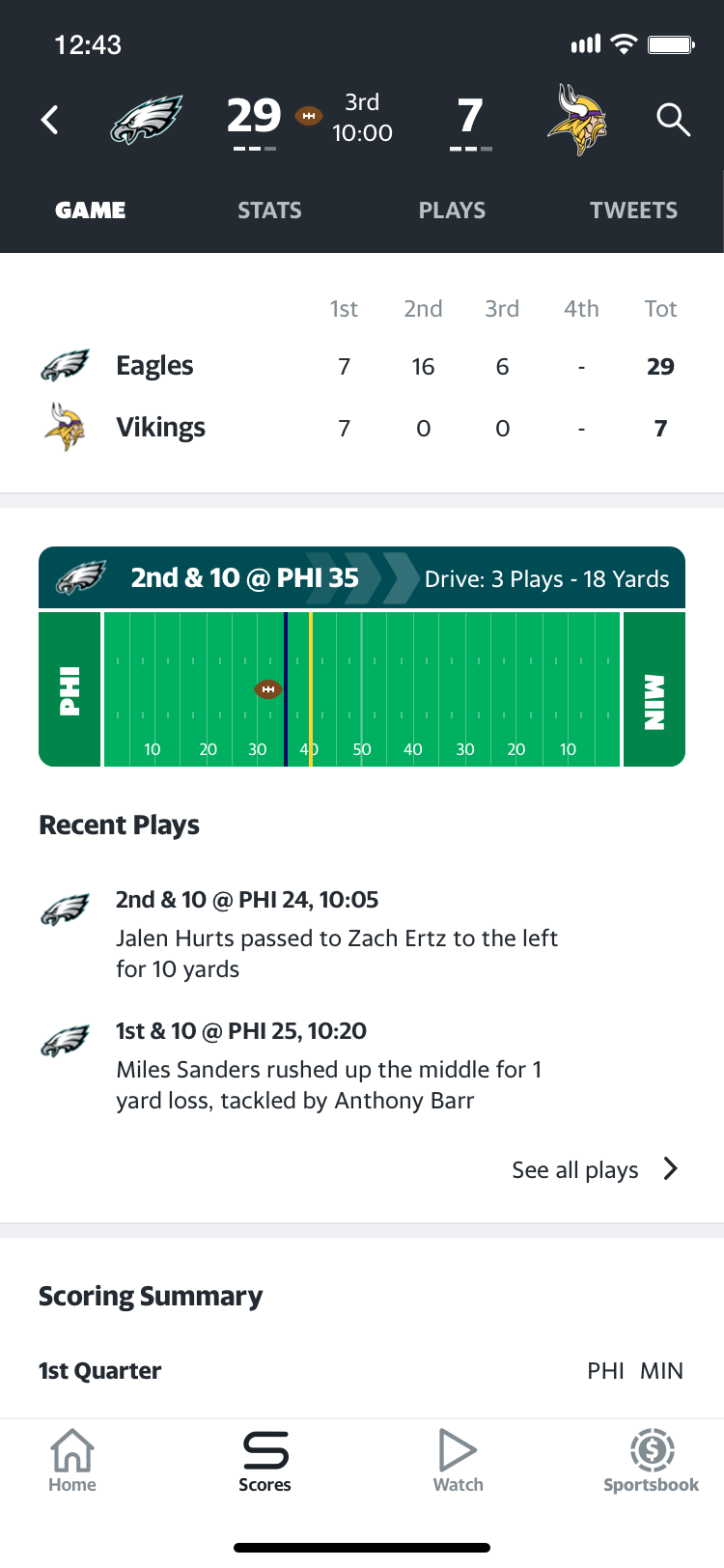A detailed screenshot of a football game score between the Philadelphia Eagles and the Minnesota Vikings is displayed. The Philadelphia Eagles are positioned on the left-hand side with a score of 29, while the Minnesota Vikings are on the right-hand side with a score of 7. The game is currently in the third quarter with 10 minutes remaining. A football icon next to the Philadelphia Eagles' score suggests they have possession of the ball. Below the main score display, there is a horizontal menu with options labeled "Game," "Stats," "Plays," and "Tweets," where "Game" is highlighted in white, indicating it is selected. Another section below displays the breakdown of points scored by each team per quarter; in the third quarter, the Eagles have scored 6 points, and the Vikings have yet to score.